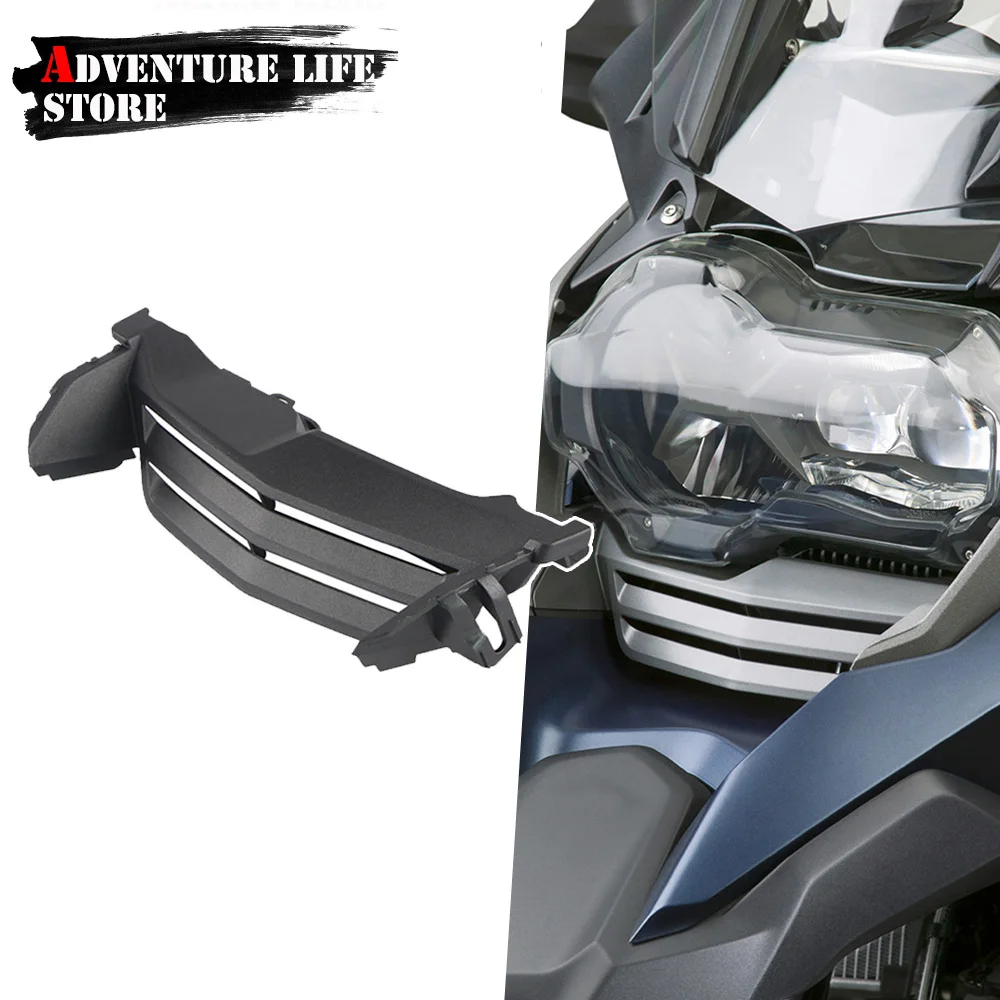The image portrays a detailed scene with a mix of graphical and photographic elements. On the top left corner is a manual drawing of a logo reading "Adventure Life Store." The "A" in "Adventure" is prominently colored red, while the remaining letters are white against a black background that appears scribbled. Below the logo, a dark gray plastic piece with three tiers is visible. On the right side of the image, there is a photo capturing the intricate interior of a car. The car parts, which seem to include pieces of the fender, grille, and possibly a headlight, are colored in dark gray, blue, silver, and white. The background on the left side of the image remains completely white, providing a stark contrast to the detailed car parts showcased on the right. Overall, the assembly of car parts and equipment, along with the distinct logo, suggests a themed composition related to automotive adventure or repair.